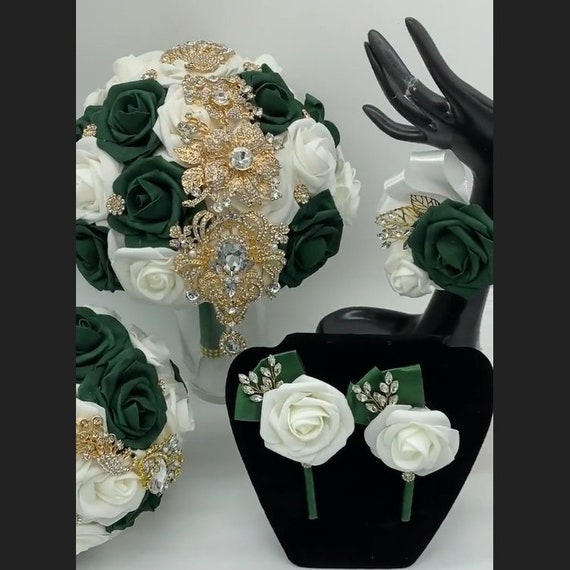This photograph features an exquisite bridal set displaying various floral arrangements and accessories, each meticulously crafted from white and emerald green satin roses. Central to the image is a large, round bouquet poised in a clear glass vase, adorned with gleaming gold and crystal embellishments that cascade down its center, complemented by small gold and crystal pins scattered among the roses. On the right, a black mannequin hand showcases a delicate wrist corsage, featuring a green satin rose, a smaller white rose, a white satin bow, and gold leaf accents. To the left, a black velvet necklace display holds two white satin roses accented with green satin leaves and sprays of crystals and gold, likely designed for pinning on the groom's and groomsmen's suits. Additionally, a smaller round bouquet of similar white and emerald roses sits prominently, suited for the bride, the bride’s mother, or a bridesmaid, also adorned with elegant gold and crystal detailing. The background of the photo is gray, flanked by black borders on either side, enhancing the display's elegance and sophistication.